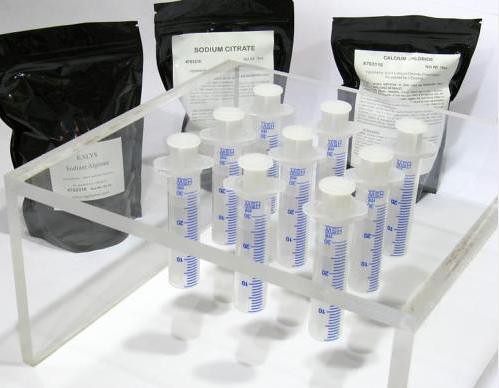The image is a detailed photograph of a medical laboratory setup. Central to the image is a clear plexiglass box housing nine syringes positioned in a clear tray. Each syringe is transparent with white tops and features blue graduated markings and numbers for measuring volume. The setup casts detailed shadows on the pristine white surface below. In the background, you can see three black plastic bags with labels. The middle bag is clearly marked "sodium citrate," while the text on the bags to the left and right is mostly illegible, although the right one seems to include the word "calcium." The entire scene is set against a white backdrop, contributing to the overall sterile and clean appearance of the laboratory environment.